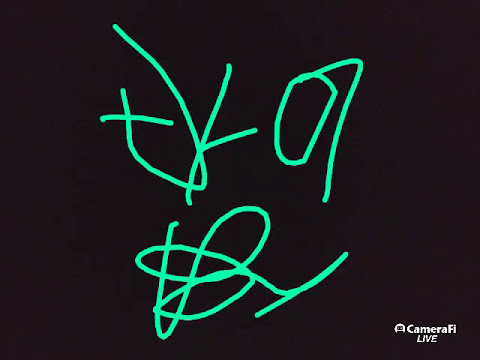In the center of the image, there is a drawing comprised of bright green, scrawled lines against a completely black background. The green lines resemble scribbled text or random, unidentifiable shapes, possibly suggesting letters like T, A, B, Y, O, J, and P. This haphazard drawing could be reminiscent of child-like or artistic doodling done on a paint program via a tablet or smartphone, where the text is difficult to interpret or read clearly. The scribbles dominate the middle of the image, possibly forming abstract designs or creative lettering. In the bottom right corner, there is a logo that reads "CameraFi Live." The overall visual gives the impression of spontaneous, creative expression, accentuated by the stark contrast between the vivid green lines and the solid black background.